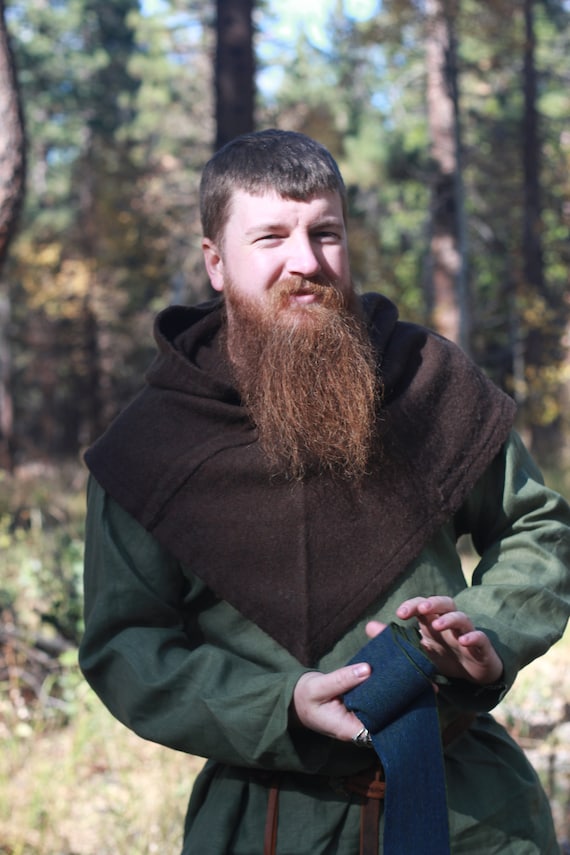The photograph captures the scene of a man, possibly a modern-day monk, standing outdoors in the foreground of a forested area. The man is central to the image, wearing a gray-green robe with a hooded, triangular-shaped upper piece that drapes down past his shoulders to his chest. He features short brown hair and a strikingly long red beard that flows down to his chest, complete with a full mustache. His attire includes a brown belt and a V-shaped collar that extends to his waist. The man is holding a long strand of blue cloth in his hands, which he is rolling together in front of him. The background is filled with out-of-focus tall grass, wild plants, and trees. The lighting suggests a sunny day, with the man squinting slightly at the camera, and a blue sky visible behind him. The overall palette of the image is composed of earthy tones including green, brown, blue, tan, and beige, blending harmoniously with the natural outdoor setting.